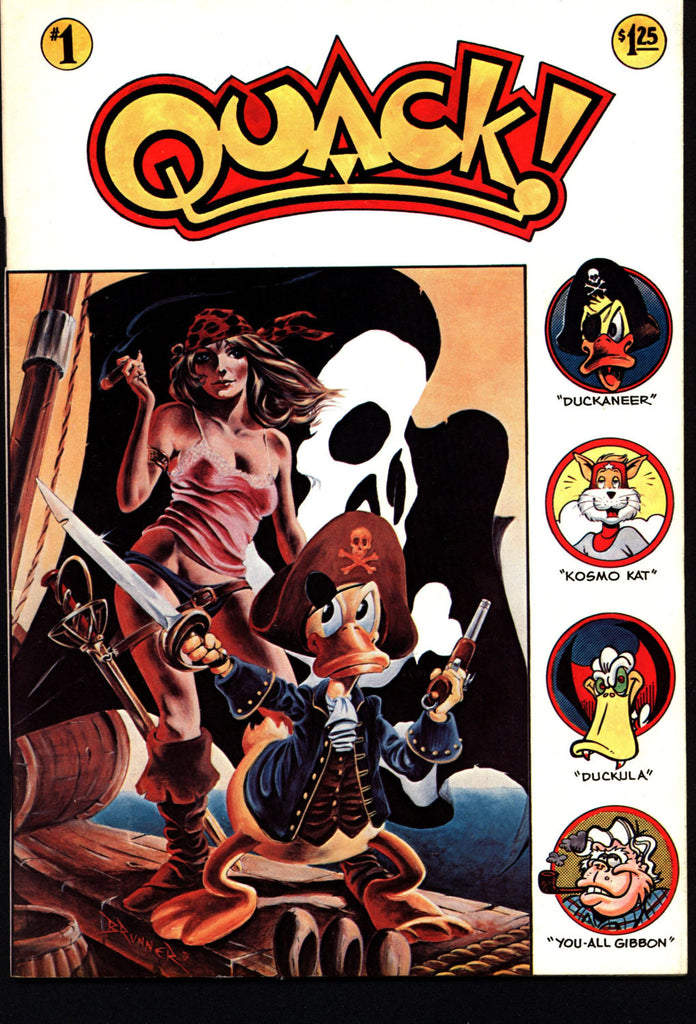This is the highly detailed cover of the premier issue of a comic book titled "Quack," sold for $1.25. The title "Quack!" is prominently displayed at the top in a highly stylized gold font, outlined first in black and then in red. The number "1" is encased in a gold circle at the top left, indicating the inaugural issue. The main illustration features a cartoonish, anthropomorphized duck dressed as a pirate captain. This duck wields a pistol in one hand and a raised sword in the other. He sports a pirate hat adorned with a skull and crossbones and an eye patch resting slightly above his left eye to reveal it. He wears a blue captain's jacket and a vest, but notably no pants.

Standing behind the duck is a pirate woman wearing a red bandana (sometimes described as leopard-print) and an eye patch over her left eye. She is dressed in a skimpy pink tank top or camisole, short shorts or a black thong that is slightly pulled down over her hip, and knee-high brown boots. The background features a large black pirate flag with a skeleton emblem.

Along the right side of the cover are four additional character illustrations. The first is another depiction of the pirate duck labeled "Duckineer." Below that is a cat named "Cosmo Kat," followed by a vampire duck with bloody fangs labeled "Duckula." The final character is a vaguely humanoid creature labeled "You-All Gibbon," who is portrayed smoking a pipe.